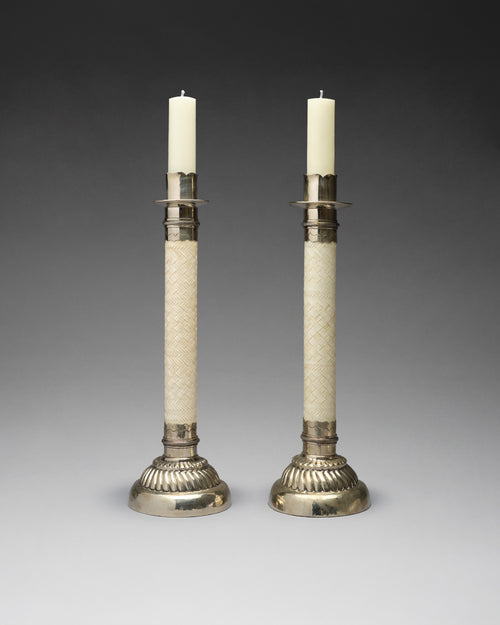This professional photograph features a pair of elegantly tall and thin beige candles displayed in ornate silver candlestick holders. The candlesticks, with their meticulously polished silver surfaces, stand on a three-layered base: a series of rings decreasing in size from a large bottom ring to a smaller top ring. The candles themselves are about a foot and a half tall, though this may be an illusion due to the smooth, professional lighting. The holder's body is of white material and features a sophisticated design, including metal bindings with silver bands and protrusions near the upper middle. At the top of each candlestick is a small ledge designed to catch dripping wax. The background of the photograph transitions seamlessly from a dark, almost black shade at the top to a light gray at the bottom, where it meets what is presumably the table surface. The candlesticks’ diameter at the base is roughly three inches and they feature intricate, ornate carvings, enhancing the elegance of the composition.